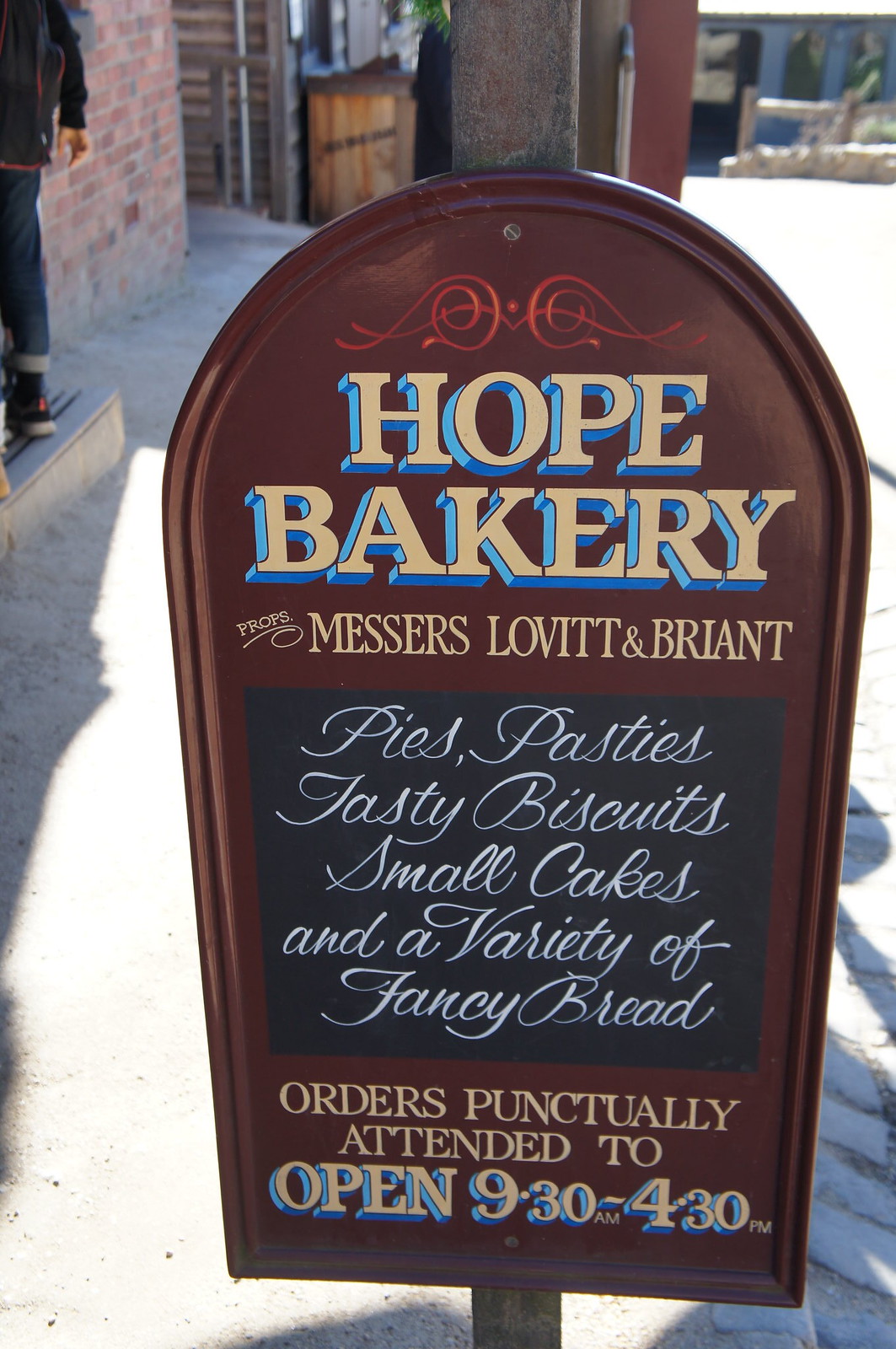The photograph captures a detailed exterior scene featuring a sign on the sidewalk in front of a red brick building. The sign, which is attached to a wooden post, is brown and appears to be made of metal, resembling a tombstone shape with a rounded top and flat bottom. At the top of the sign, a decorative red script design adorns the header. Below this, prominent tan letters with a blue border spell out "Hope Bakery." The proprietors, Messrs. Lovett and Bryant, are listed beneath this in similar tan letters. The central section of the sign contains a blackboard-like square with neatly printed white cursive that reads: "Pies, Pastries, Tasty Biscuits, Small Cakes, and a Variety of Fancy Bread." At the bottom, in tan letters, an assurance is given: "Order Punctually Attended To." The sign also conveys the bakery's operating hours, "9:30am to 4:30pm," in the same tan and blue bordered style. The image also captures part of the surrounding area, including cement pavement and a glimpse of a person wearing dark clothing in the background.